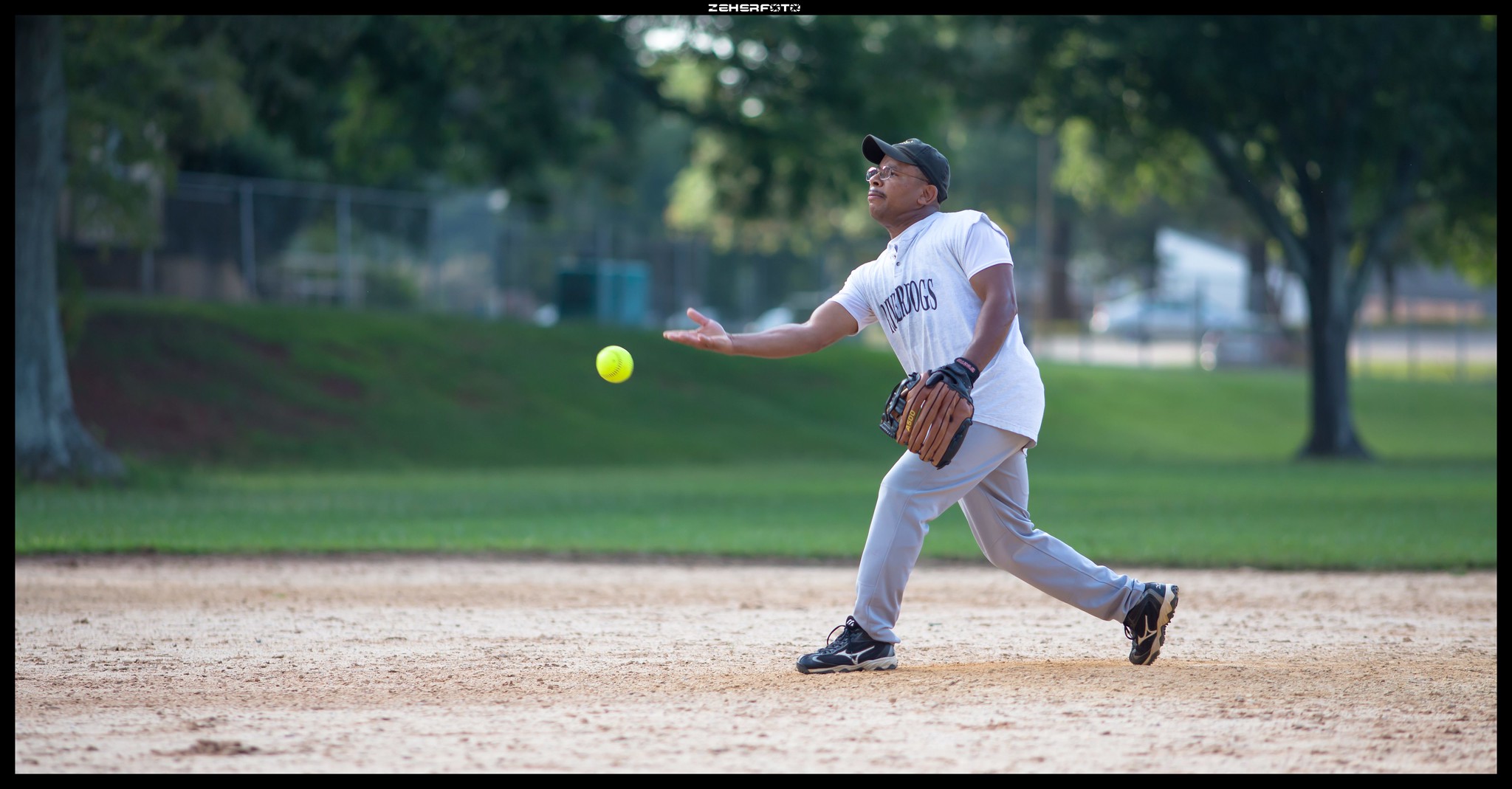In this daylight action shot, an African American man is captured in mid-throw, his right arm fully extended as he pitches a yellow softball in a park. He is dressed in a white short-sleeve shirt with blue lettering, gray pants, and black sneakers with white accents. The man, who sports glasses and a mustache, also wears a blue baseball cap and a glove on his left hand. The scene is set on the dirt mound of what appears to be a baseball diamond. The background reveals a green field dotted with trees and a blurred metal fence, suggesting an enclosed park setting. The sun casts its rays over the lush surroundings, adding to the dynamic atmosphere of the moment.